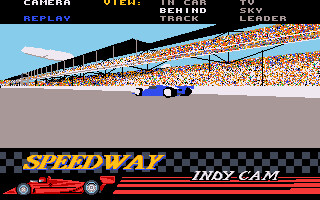The image is a detailed screenshot from a computer game, depicting a vibrant racing scene. At the very top, there is a black border with various camera view options labeled in different colors: "Camera" in white, "Replay" in blue, "View" in yellow, "In Car" in gray, "Behind" in white, "Track" in gray, and "TV Sky Leader" also in gray. Below this header, the main focus of the image is a realistic racetrack under a bright blue sky. The grandstand, stretching across two stories, is packed with a multicolored audience, represented by tiny dots of red, white, blue, and yellow, suggesting the presence of fans. The gray roadway in front of the grandstand features a blue race car prominently on the track. At the bottom of the image, a black and gray checkered section prominently displays the word "Speedway" in yellow. Just beneath this checkered area, there is a red section lined with red lines, bearing the label "Indy Cam" in white. To the left of these lines, a red sports car appears to be driving away to the left, adding dynamic motion to the scene.